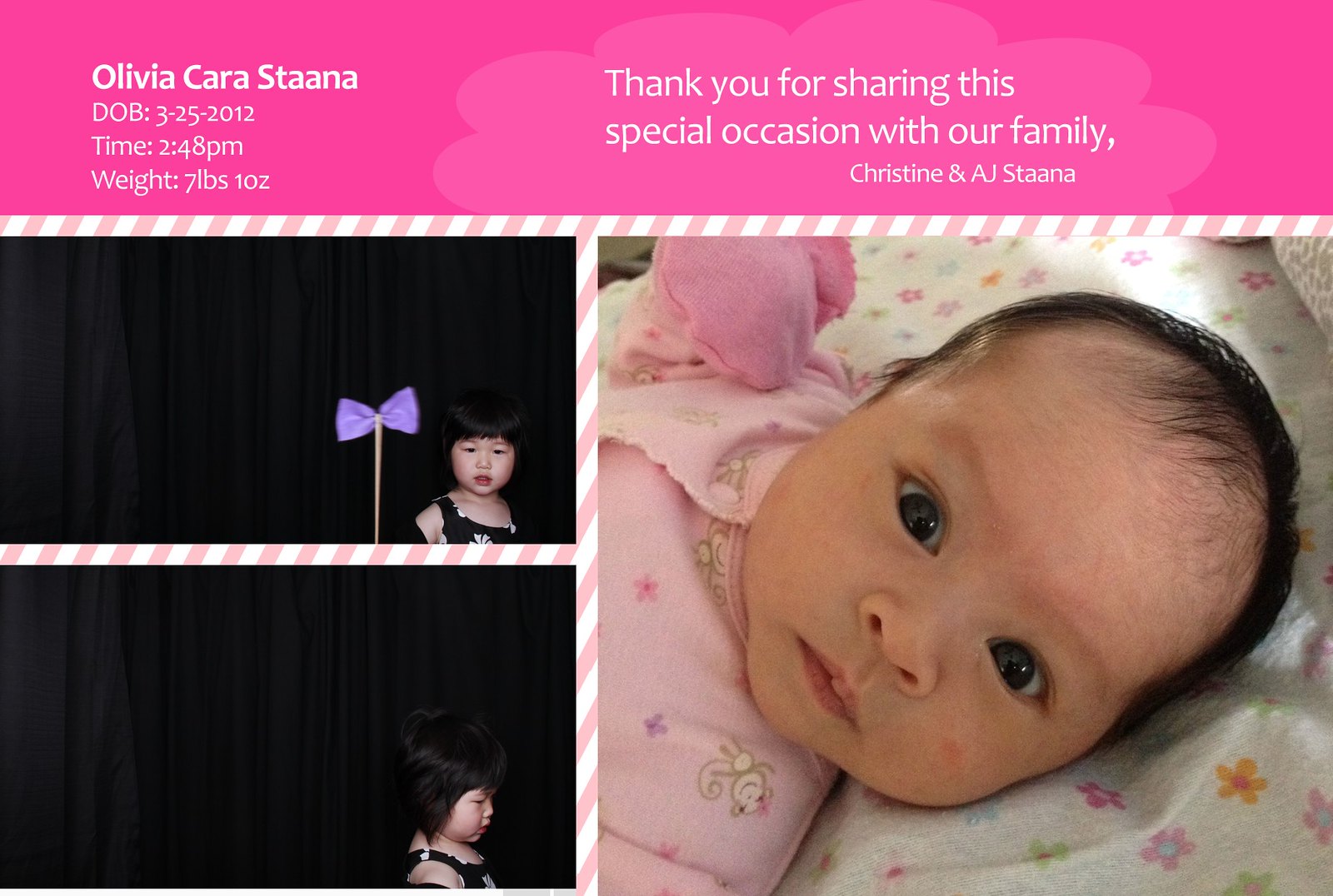A beautifully designed announcement card features a full-color photograph of a baby named Olivia Cara Stana, born on March 25, 2012, at 2:48 p.m., weighing 7 pounds and 10 ounces. The card has a pink border at the top with white print detailing Olivia's birth information and a heartfelt message: “Thank you for sharing this special occasion with our family, Christine and AJ Stana.” The card's layout includes three photographs: one large image on the right showing a newborn Olivia in a pink onesie adorned with a little monkey, pink gloves, and lying on a white blanket with colorful flowers, her black hair and bright eyes gazing up at the camera. On the left, there are two smaller photographs of an older girl, likely Olivia as a toddler. In the top photo, she is holding up a pinwheel and facing the camera against a dark background. In the bottom photo, she is looking to the right. These images collectively celebrate Olivia's arrival and the joy she brings to her family.